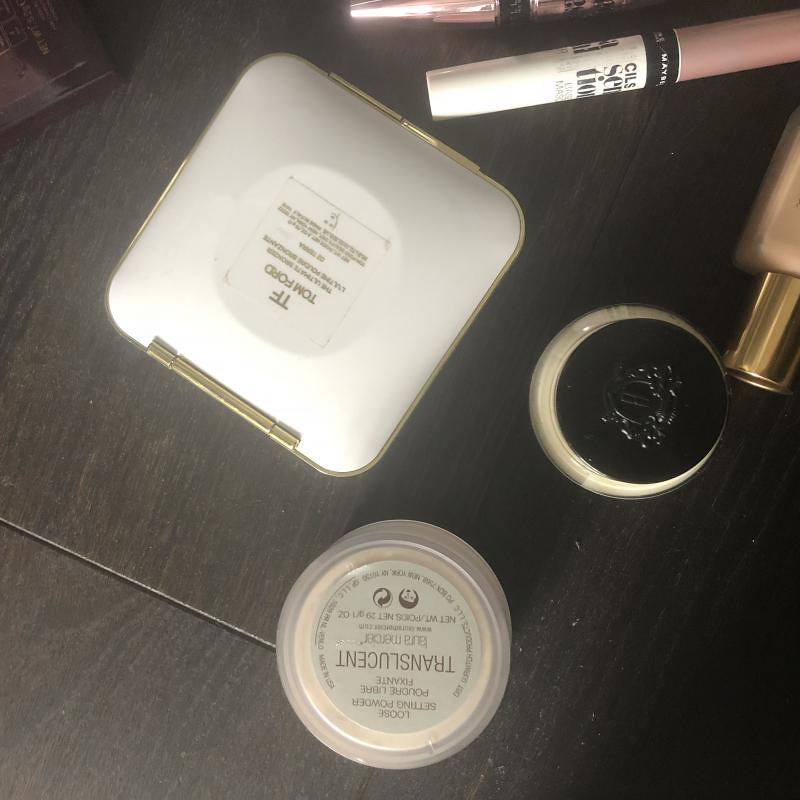In the photograph, we see an assortment of makeup products carefully arranged on a dark wood table. The centerpiece is a square compact, distinguished by its white base and gold trim around a hinge and a small clasp. The compact is identified as a Tom Ford product, emblazoned with the brand’s initials, "TF". Next to the compact lies a long white tube with a beige cap and black strap, partially revealing the brand "Maybelline". This tube appears to be either eyeliner or mascara. Among the items is also a container of loose setting powder, labeled as translucent, likely used for blending makeup and covering blemishes. Another notable item is a small round jar with a black lid. The careful placement of these products on the richly textured wooden surface evokes a sophisticated and meticulous aesthetic.